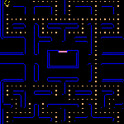The image is a small, one-inch square depiction of a game reminiscent of Pac-Man, devoid of characters like Pac-Man or ghosts. The game screen features a black background with a grid-like maze composed of glowing blue lines. Scattered across this maze, there are yellow or gold circle-like pellets, resembling the dots from Pac-Man. At the very center of the image, there is a blue-outlined rectangle with a bright pink bar at its top. Additionally, a slightly triangular cluster of tiny yellow lights can be seen in the upper left-hand corner. The overall aesthetic is reminiscent of an old-fashioned computer game, with elements that also evoke the appearance of a lit-up computer chip.